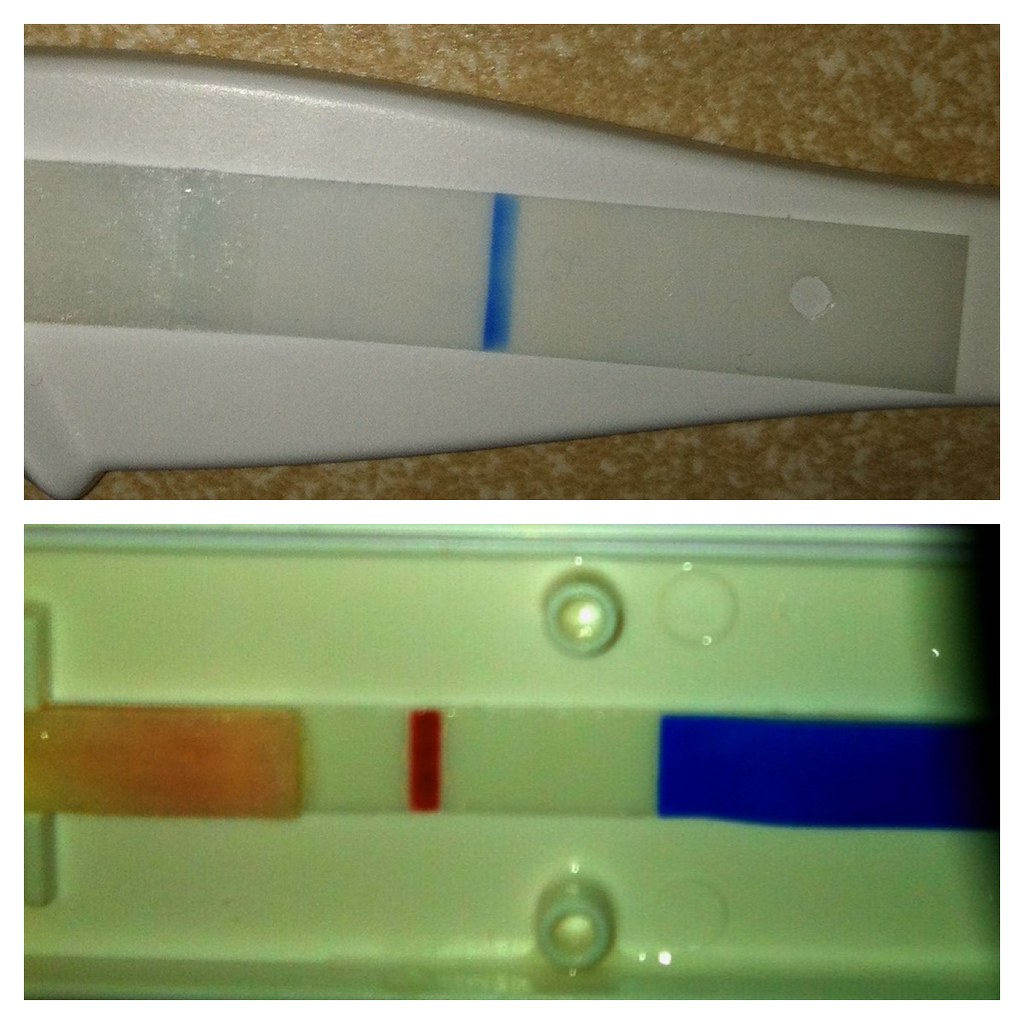This image features two pregnancy test sticks, each depicted in separate photographs. The top photograph showcases a white, oblong-shaped pregnancy test made of a solid, plastic material. Prominently displayed in the middle of the stick is a blue line within a long, rectangular, translucent section. To the right of this section, there's a small circular area where the translucent material is etched out. The item is placed on a counter with a yellow and white, somewhat messy pattern.

The bottom photograph presents a different pregnancy test, likely from another brand, characterized by a more rectangular shape. The left side of this test shows a pinkish-yellow bar, while the right side features a blue bar. Both bars are rectangular and run horizontally across the stick. Between these colored bars is a white, rectangular, translucent section with a solid red line running vertically through the middle. The blue line in the top test suggests a positive result, indicating pregnancy, while the solid red line in the bottom test suggests a negative result, indicating that the woman is not pregnant.